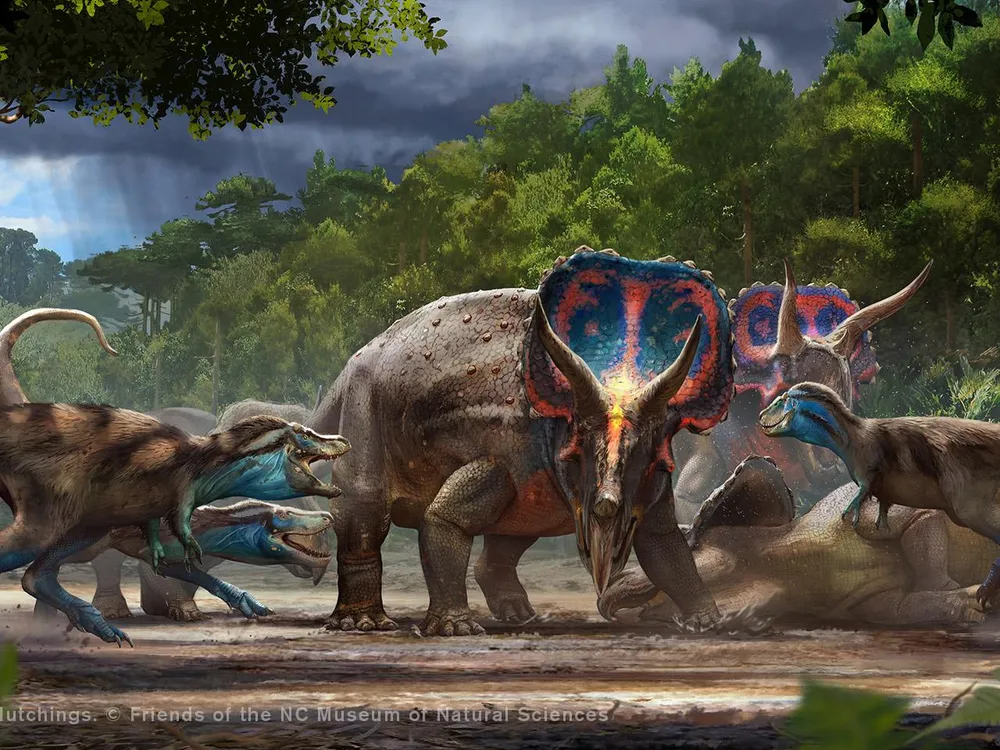The painting, credited to the "Friends of the NC Museum of Natural Sciences" in white letters at the bottom, vividly portrays a dramatic prehistoric landscape. Dominating the center is a large dinosaur with prominent horns and a distinctive blue and red design on its back, resembling a Triceratops. This creature stands on all four sturdy legs, facing the viewer with a big horned plate above its narrow skull. Nearby, a second, similar dinosaur with long horns and the same striking blue-red coloration is seen in the background.

On the left of the central creature, two smaller, raptor-like dinosaurs with open mouths and visible teeth are seen. These creatures have short front legs and long, blue back legs, giving them a somewhat rat-like appearance with lizard-like heads. One dead dinosaur lies on its side in the center foreground, with another dinosaur, bearing a blue head, standing over it with its front feet.

The scene is set on a dirt ground, with a backdrop of tall forest trees under a gloomy, gray sky that threatens rain. The atmosphere, with dense vegetation in the distance and dark clouds above, adds to the tension and drama of this vividly rendered prehistoric tableau.